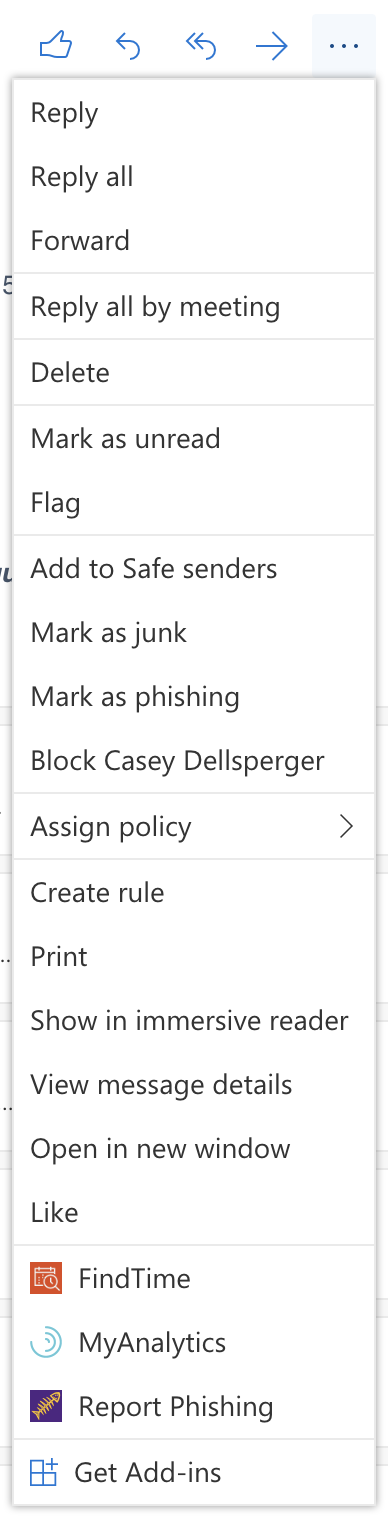This image depicts a segment of an email application's interface, specifically focusing on a drop-down menu. The drop-down menu occupies a small portion of the screen, with the rest of the interface beyond view. It is encapsulated in a thin, elongated gray box with multiple options that are left-aligned. 

Above the menu, there are several functional icons: a thumbs-up, a reply button denoted by a single arrow, a reply-all button illustrated by a double arrow, a forward button with a right-facing arrow, and three dots indicating additional options. 

The drop-down menu itself is structured into several sections, each separated by a gray horizontal bar. The first section consists of three options: "Reply," "Reply All," and "Forward," all listed vertically. Below this, there's an option to "Reply All by Meeting" followed by another gray bar. Next, there is the "Delete" option, succeeded by another gray bar. 

The following section includes: "Mark as Unread" and "Flag," followed by another gray bar. Below this, four more options are listed vertically: "Add to Safe Senders," "Mark as Junk," "Mark as Phishing," and "Block Casey Delsberger," each divided by a horizontal bar. 

Further down, there is an option labeled "Assign Policy" accompanied by a right-facing caret, then another separating horizontal bar. The next section lists: "Create Rule," "Print," "Show in Immersive Reader," "View Message Details," and "Open in New Window," all vertically aligned, followed by another gray bar. 

At the bottom, there are three options each paired with an icon: a red calendar icon next to "Find Time," a blue multi-circle icon labeled "My Analytics," and a fishbone icon on a black background identified as "Report Phishing." Beneath this last section, a horizontal bar is present with the text "Get Add-ins" adjacent to three small boxes and a plus sign on the left.